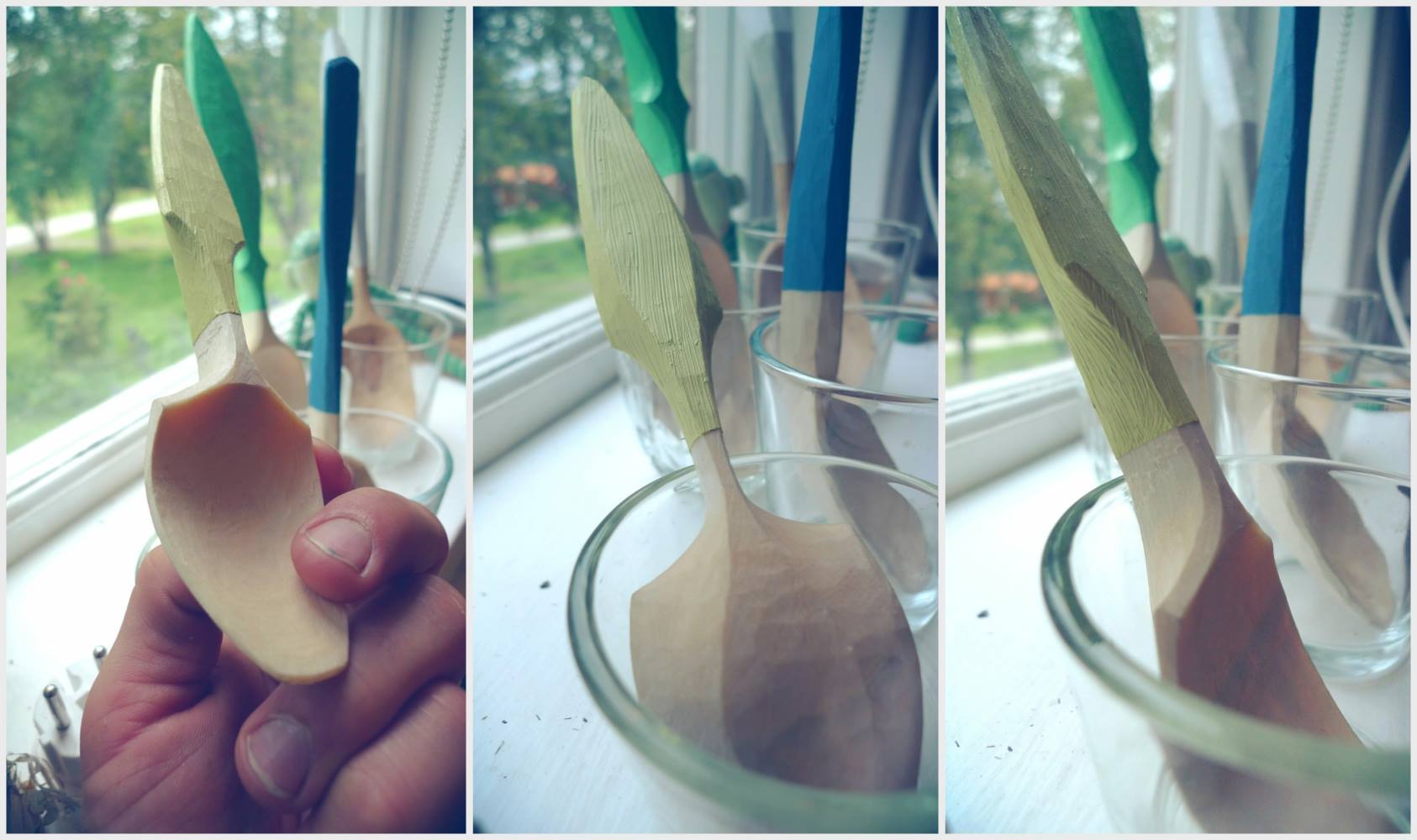A landscape-oriented image showcases a meticulously hand-carved wooden spoon through three distinct, side-by-side photographs, each providing a different angle of the intricate craftsmanship. In the first photo on the left, a man's hand, set against a garden backdrop, delicately holds the spoon by its concave part, revealing its smooth, front side. Behind this central spoon, similar utensils can be spotted, hinting at a collection. The middle photo displays the spoon placed in a bowl, the back of the spoon facing the viewer, offering a different perspective. Lastly, the third photo features a side profile of the spoon, again in the bowl, giving a clear view of its elegant curvature. All photos are consistent with varying lighting and the serene, natural setting seen in the background, highlighting the artisan’s attention to detail and the spoon's versatile beauty.